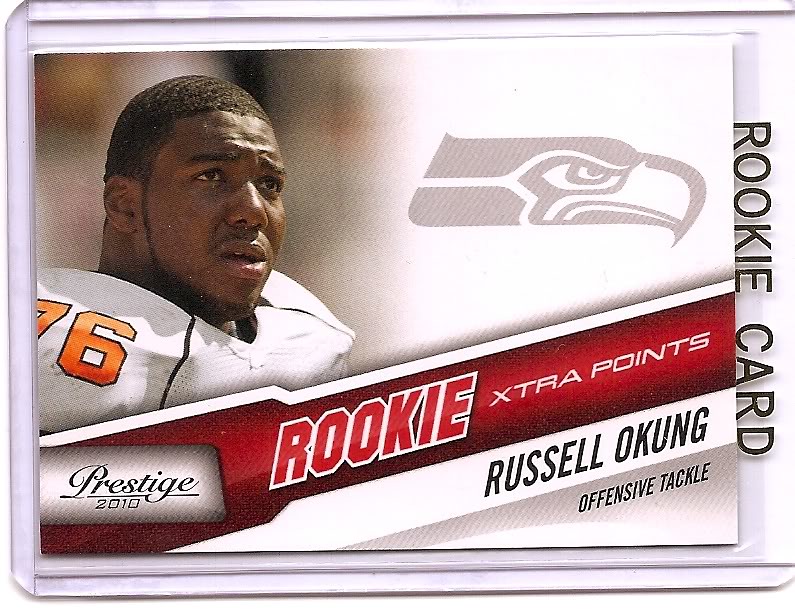This image reveals a rookie card for an American football player, prominently featuring text and imagery that highlight the player's details and the card's stylistic elements. The player, an African-American man, is depicted with short hair, a closely shaved beard, and sideburns running down to his beard. He wears a white jersey with the number 76 in yellow on his right shoulder and appears to be looking into the distance. The card includes an eagle logo in the top right corner and a red diagonal banner running from the bottom left to the middle right, stating "ROOKIE" in white outlined letters, followed by "XTRA POINTS" in black text.

Below this banner, there's another white banner with the player's name, "RUSSELL OKUNG," spelled out in black capital letters. Positioned directly underneath, in smaller font, is the player's position, "Offensive Tackle." On the bottom left corner of the card, the text "Prestige 2010" is displayed, indicating the card's edition. Vertically aligned on the right edge of the card, the text "Rookie Card" is printed in black. The card appears to be housed within a protective plastic sleeve, suggesting care and preservation for this collectible item.